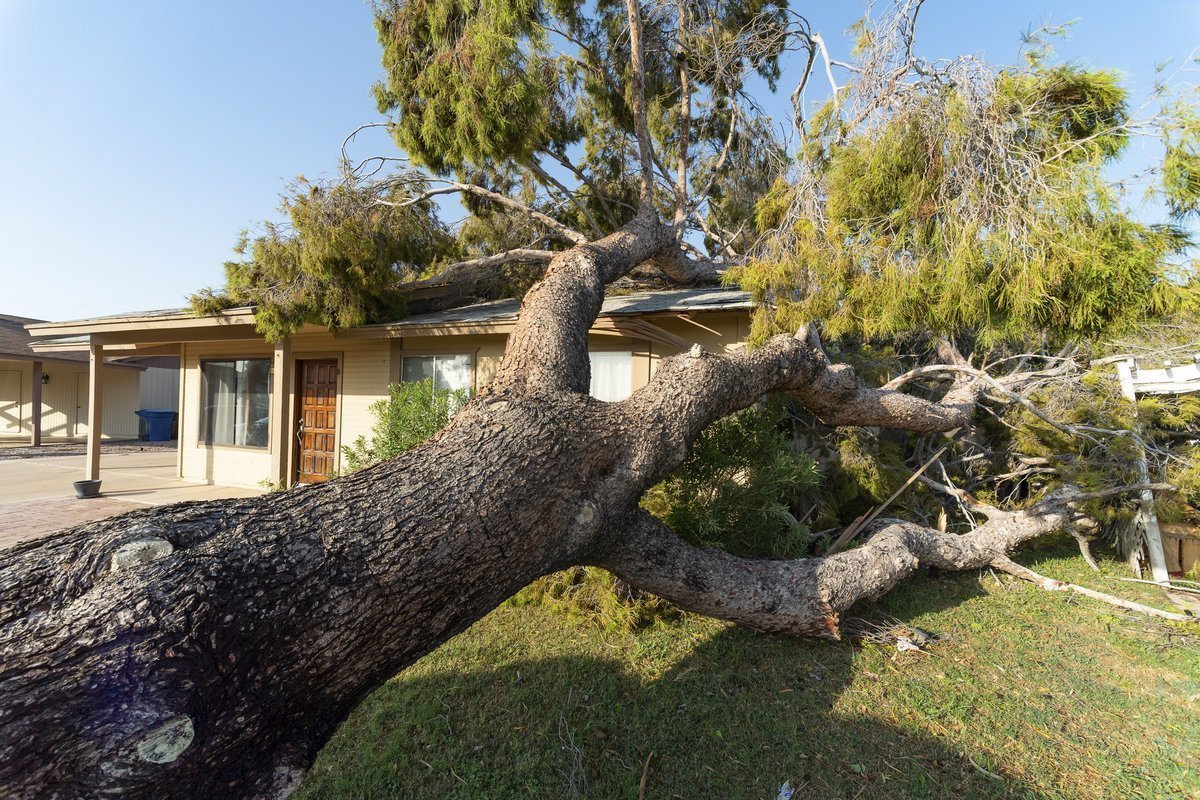The image depicts a large, uprooted tree that has fallen onto a one-story, mid-20th-century ranch-style house, possibly located in a desert region like Arizona, based on the clear, cloudless blue sky and the type of pine tree. The tree, with its thick grayish-brown trunk and three substantial branches laden with bright green leaves, rests heavily on the roof of the house, potentially causing significant damage, especially to the right side and potentially a shed or outbuilding. Despite the tree impacting the house, certain elements like the large wooden front door, side windows, and a carport remain intact, suggesting the damage might be limited to specific areas. The house, painted in an off-white color with a minimally sloped roof, sits amid green grass, emphasizing the context of the surrounding yard. The scene is lit by daylight, casting shadows and highlighting the contrast between the devastation caused by the fallen tree and the tranquil, sunny weather.